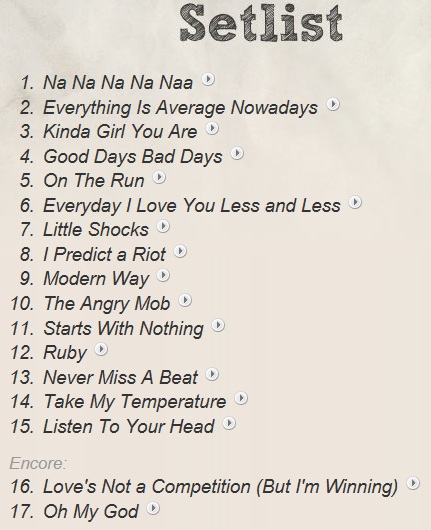The image features a rectangular, off-white sheet of paper with a slightly drab appearance. At the top, slightly off-center to the right, in large, filled-in black letters, it reads "SETLIST," although the word is misspelled as "SETLAST." Below this heading is a list of 17 songs, all typed in dark gray, left-justified text.

The setlist starts with "1. Na-na-na-na-na" and continues down to "15. Listen to Your Head." Following this, in a smaller gray text, the word "ENCORE" introduces the final two tracks, "16. Love's Not a Competition (But I'm Winning)" and "17. Oh My God."

Next to each song title, there is a small white circle containing a right-facing arrow, resembling a play button, giving the impression that the list might function interactively, as if clicking the arrow could play the song. The paper's background is a light, whitish-gray color, and the entire document has a somewhat scruffy, scanned appearance, even though it could just be a printed sheet. The layout is straightforward, emphasizing the raw and minimalist design.